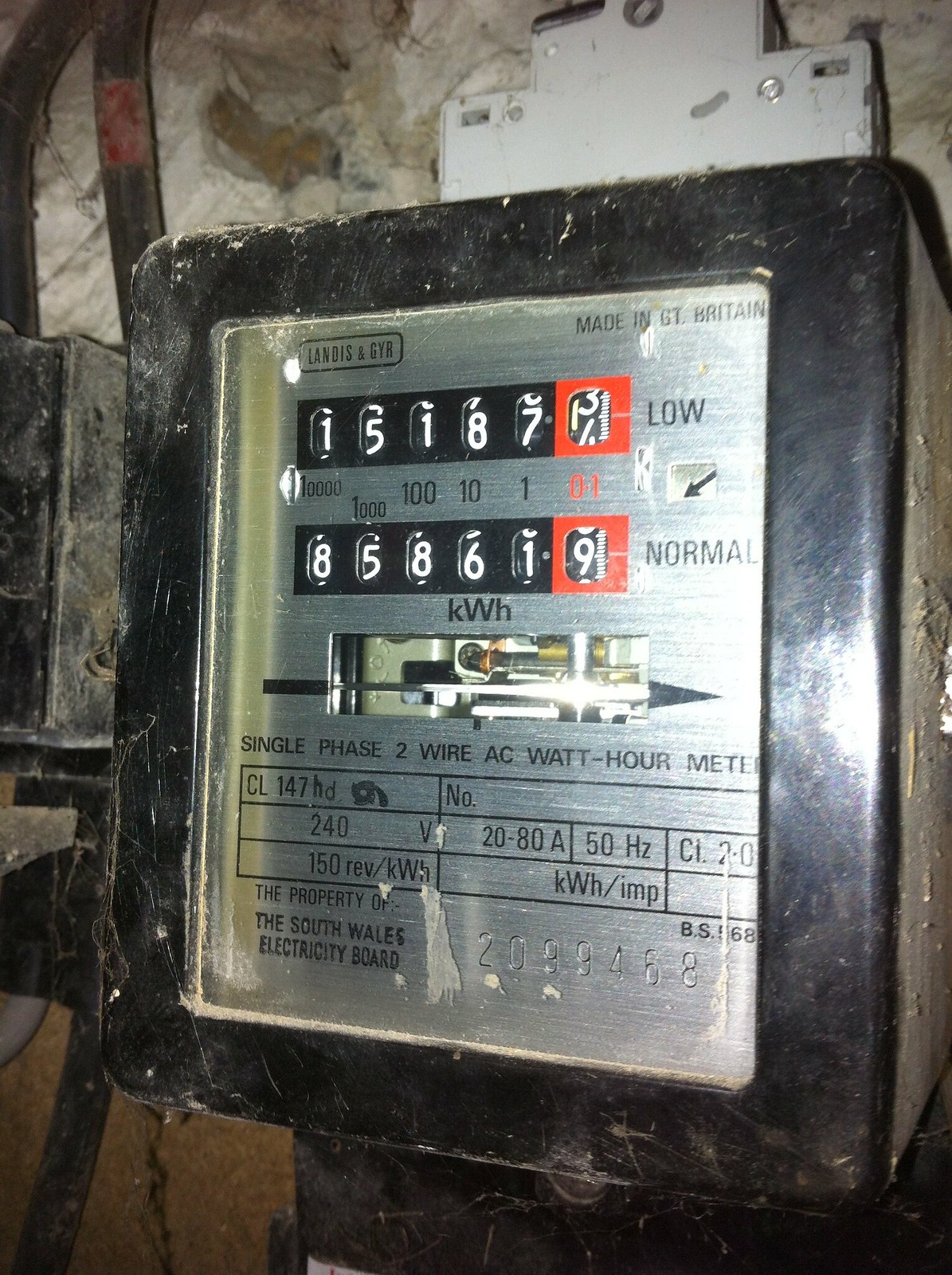The photograph depicts the inside of a meter cupboard featuring an old, industrial-looking, black meter with a silver panel marked “Landis and Gyr” in the top left corner and “Made in GT.Britain” on the top right. Behind a clear plastic cover, a series of electrical gauges and wires are visible. The first black panel displays the number 15187, while adjacent, within a red segment showing a value between 3 and 4, the label “Low” appears. Below this, a secondary black panel reads 85861, with a red section marked “Normal” displaying the number 9. Additionally, in the bottom right-hand corner, there is a code, 2099468. The apparatus, possibly related to a single-phase two-wire AC watt-hour meter, is nestled within a black box, indicative of an industrial environment, potentially underground.